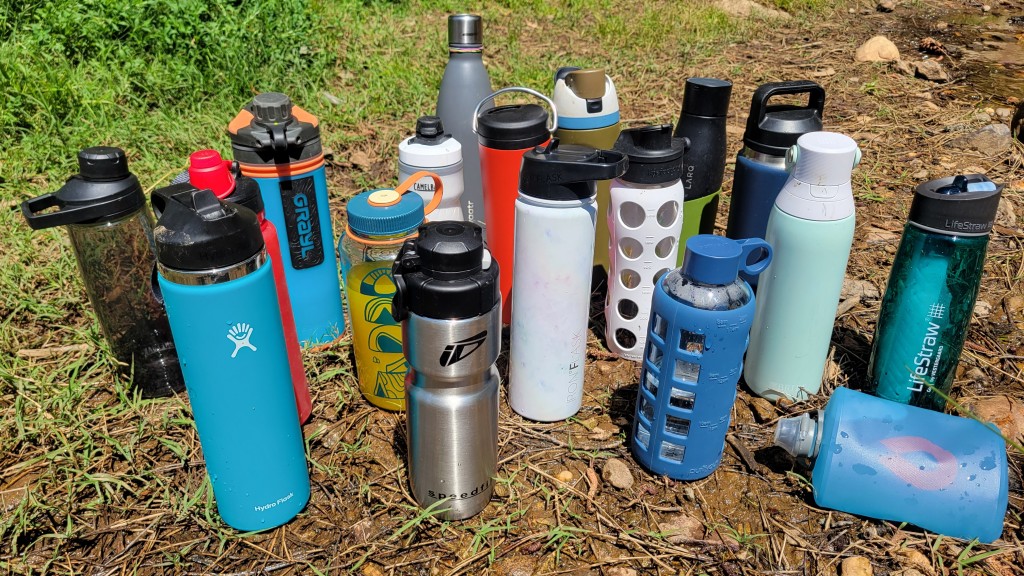The image is a detailed color photograph, shot in landscape orientation, depicting a collection of 19 various water bottles scattered on the ground, which is a mix of dirt, rocks, and sparse grass. The vantage point is from a low angle, slightly looking down. The water bottles are a diverse assortment in size, shape, color, and brand, with notable mentions including Life Straw, Hydro Flask, and Gravel bottles. They range in colors from gray, blue, red, to see-through green and black, and some even have unique designs such as a blue flask-shaped bottle with a pink circle that's laying on its side in the bottom right corner of the image. Most of the bottles are standing upright, except for the aforementioned flask. The ground also features twigs and sparse greenery, with a dirt trail visible in the upper right corner and more grass on the upper left. One bottle notably seems to contain orange juice, adding an unusual detail to the collection focused on hydration during an outdoor event.